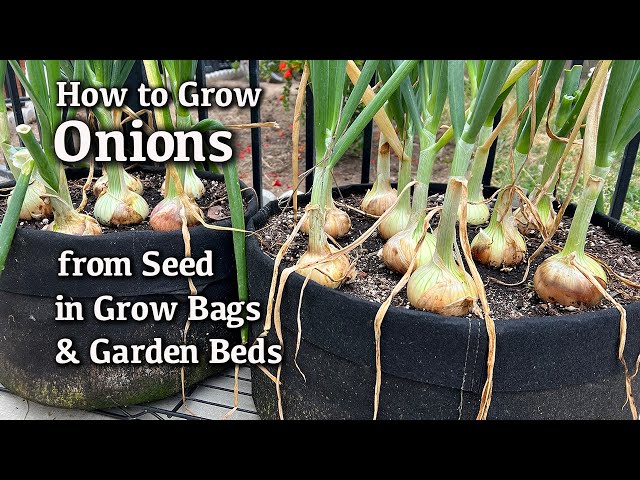The image features two large, black cloth grow bags filled with dark soil and sprouting onions. The onions have papery bulbs that protrude from the packed dirt, with tall green stems rising above. In the background, a garden with a fence-like structure and what appears to be strawberries growing on vines can be seen. The scene is set outdoors, likely on a wooden surface, under an overcast sky. In the top left corner of the image, white text reads: "How to Grow Onions. From seed, in grow bags, and garden beds."